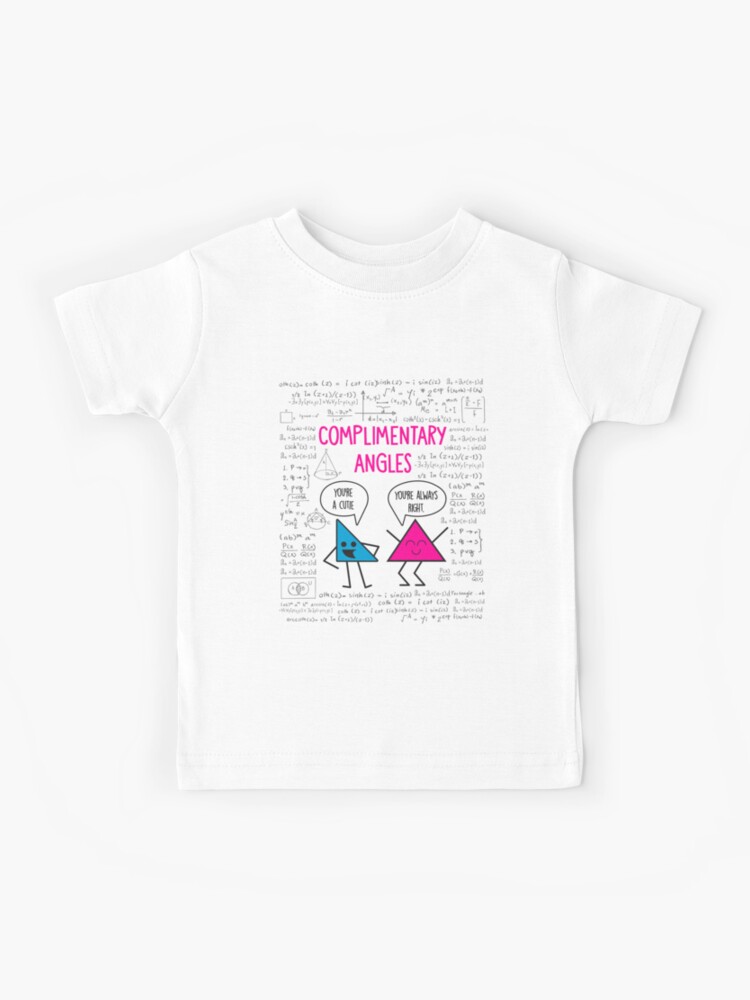This image showcases a child’s white, short-sleeved t-shirt, displayed on a white background, likely a mock-up for a web store. In the center, the shirt features a playful math-themed design in a rectangular layout. The prominent text in big pink letters reads "Complementary Angles." Below, two animated triangles with faces and limbs engage in a humorous exchange. The blue right-angle triangle, hands on hips, says, "You're acute," in a speech bubble. In response, the pink equilateral triangle replies, "You're always right." The background is adorned with faint, unreadable writings that resemble math problems, adding to the academic theme. Overall, the design makes for an adorable and educational children’s shirt.